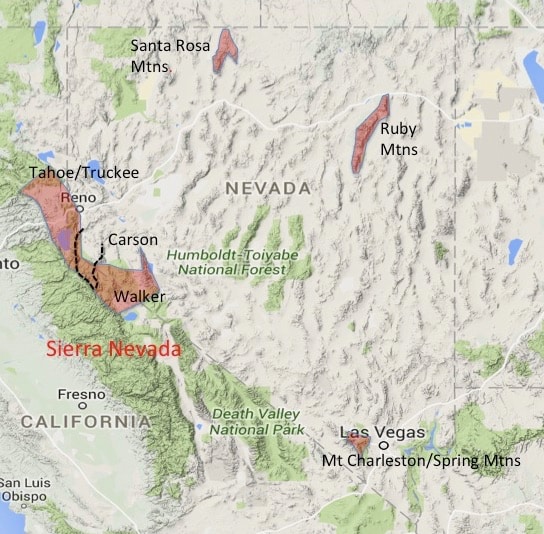This image is a detailed topographical map of Nevada, vividly showcasing various natural landmarks and geographic features. The map prominently highlights the mountainous regions with the Santa Rosa Mountains in the upper left corner and the Sierra Nevada mountain range extending through the middle left, down towards the central and lower parts. The Ruby Mountains are located towards the top, and the Humboldt-Toiyabe National Forest is centrally positioned. Major landmarks like Death Valley National Park are outlined in tan and labeled in green, while Las Vegas and the adjacent Mount Charleston Spring Mountains appear in the lower right. Additional prominent mountain ranges such as the Sierra Nevadas are marked in red, creating a clear, textured distinction between different elevations and terrains. The state of Nevada is written in the middle of the map, with surrounding states, including parts of California and Utah, also labeled. Cities like Reno and Carson are marked in black, adding to the comprehensive detail of the map. The entire map effectively uses color and texture to indicate elevation and terrain differences, emphasizing Nevada's diverse topography.